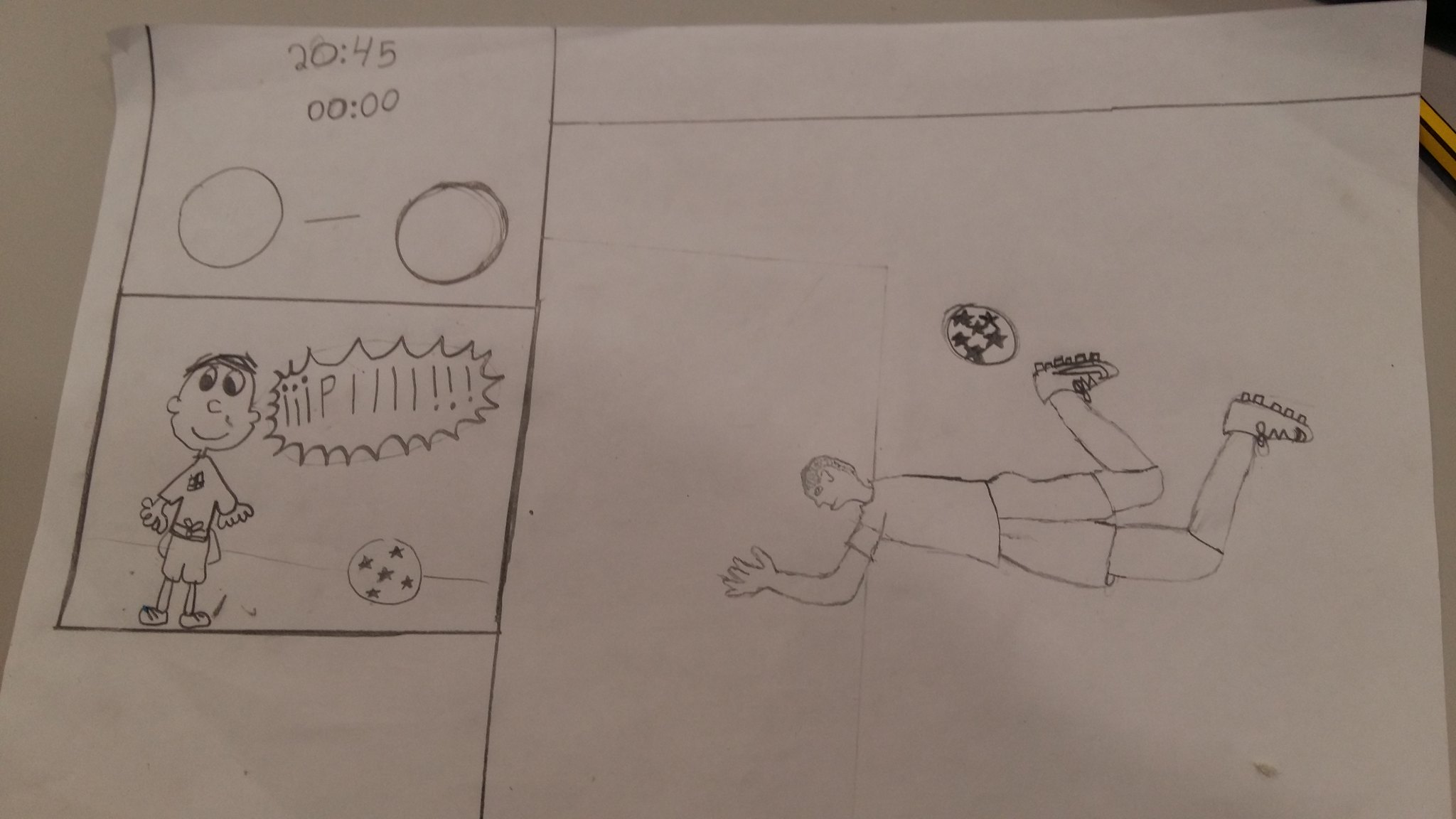This image depicts a hand-drawn scene of a soccer match, evocative of a child's imaginative artwork. The central figure is an exaggerated and disproportionate soccer player, prominently larger on the right side of the drawing. The player is sprawled on the ground, displaying a disproportionately large arm and head, and notably large legs. He is captured in mid-action, kicking a soccer ball adorned with stars using his left leg.

On the opposite side of the scene, another soccer player is depicted with a comically silly face, seemingly yelling "pee." This character lacks a neck, and their hands are humorously drawn with too many fingers. The player's pockets are oddly positioned on the outside of their attire, adding to the whimsical nature of the artwork. A second soccer ball, also featuring stars, appears in the image.

Above the characters, there are enigmatic annotations that read "20..45" and "0 0..0 0" followed by a cryptic "0 a ball minus a ball." The entire drawing is rendered in pencil, with visible eraser marks indicating corrections. The paper rests on a brown surface, likely a table, and a pencil lies on the right-hand side of the image.